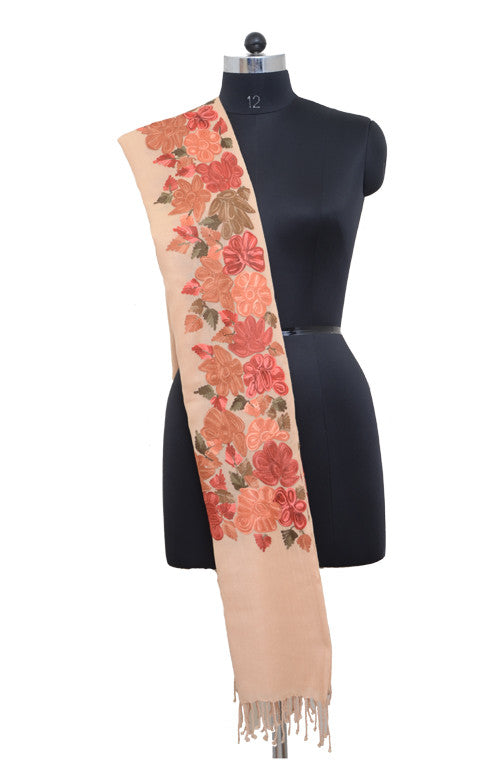The photograph showcases a black felt mannequin centered against a white background. The mannequin, which is headless, armless, and truncated at the waist, prominently features the number "12" in silver on its neck. Above the neck is a small metallic area topped with a black ball. Draped over the mannequin's left shoulder is a long, tan scarf adorned with a vibrant floral print, primarily in shades of pink and red. The scarf, ending in delicate tassels, nearly obscures the mannequin's supporting silver bar as it extends down its side. The floral pattern covers about 70 percent of the scarf, creating a striking contrast against the neutral tone of the fabric.